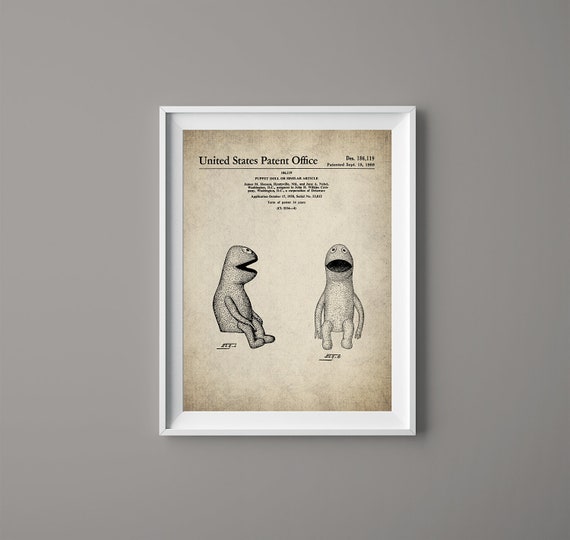The image shows a white picture frame hanging on a stylishly modern, lightly grayed wall, possibly in an updated California or Las Vegas apartment. Within the frame is a faded, yellowed tan paper, featuring a detailed illustration and several lines of text. The heading at the top of the paper reads "United States Patent Office," accompanied by an illegible date from December. Beneath the title are rows of small, unreadable text, likely detailing patent specifics. The centerpiece of the document includes two black-and-white illustrations of a character resembling a Muppet or a puppet, one oriented sideways and the other facing forward. The figure has features akin to popular Sesame Street characters like Kermit, Grover, or Bert and Ernie, and it appears unclothed, with visible arms and legs.